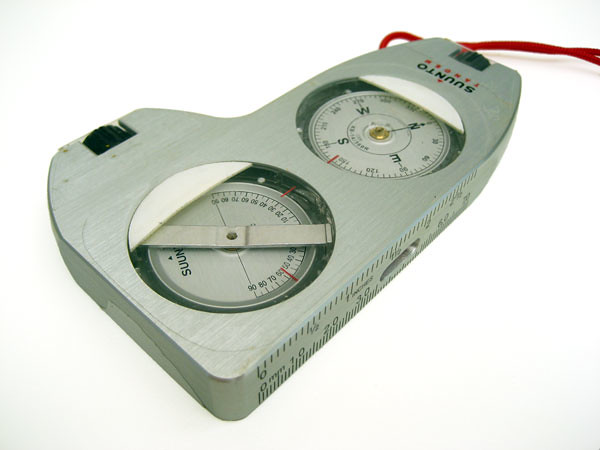This image features a precision measuring device likely used for navigation or surveying tasks. The device is made of metal and resembles the shape of a boot. Protruding from the base is a prominent red wire. At the toe section of the boot, there is a black turn knob, suggesting a part that may be adjusted or calibrated.

At the base of the device, the brand name "SUUNTO" is prominently displayed, with some unreadable red lettering beneath it. This name indicates that the device is manufactured by Suunto, a company known for creating precision instruments. Another turn knob is located towards the heel of the 'boot,' adding to the functional aspects of the instrument.

The side of the device is marked with an etched ruler, featuring a series of notches and numbers, useful for accurate measurements. On the flat top portion of the boot-like design, there are two circular dials embedded within. The first circle contains a compass, clearly marked with the cardinal directions—N, S, W, and E—and surrounded by a ring of numbers in black, which likely aid in precise navigation.

The second circular dial displays a series of numbers ranging up to 90, yet its specific function remains unclear. This dial, like the compass, hints at the device's complex functionality, possibly for measuring angles or other navigational data.